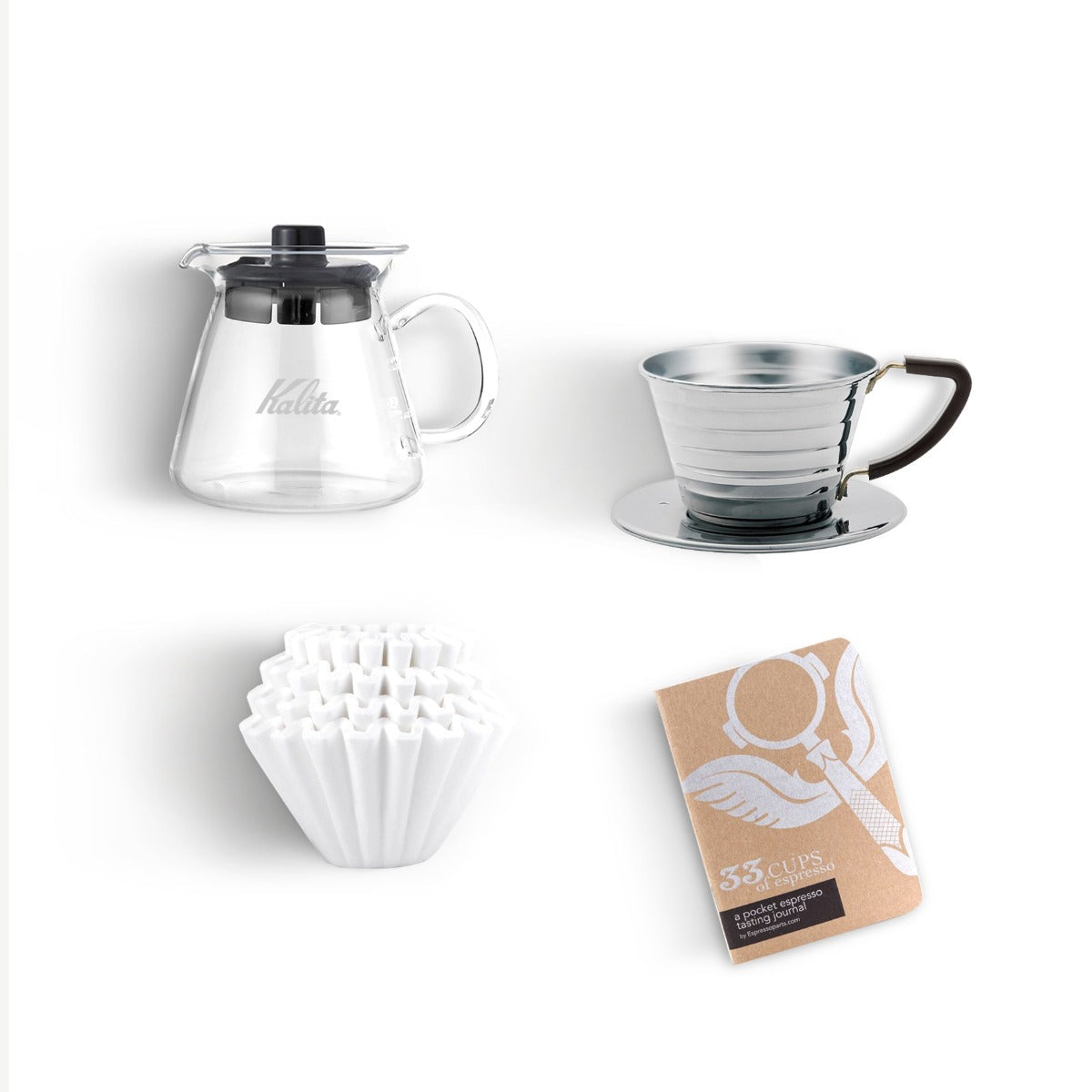The image, set against a solid white background, displays four distinct coffee-making items arranged in a grid: top left to right and bottom left to right. In the upper left, there's a glass carafe marked with the brand "Kalita" on its side, featuring a clear handle and topped by a deeply inserted black plastic stopper. To its right is an aluminum coffee cup with striped indentations and a black handle, resting on a matching aluminum saucer. The bottom left showcases a tightly stacked set of old-fashioned white, crinkly round coffee filters meant for a drip coffee maker. Finally, the bottom right shows a brown package resembling a journal titled "33 Cups of Espresso: A Pocket Espresso Tasting Journal," adorned with white graphics of a winged creature.